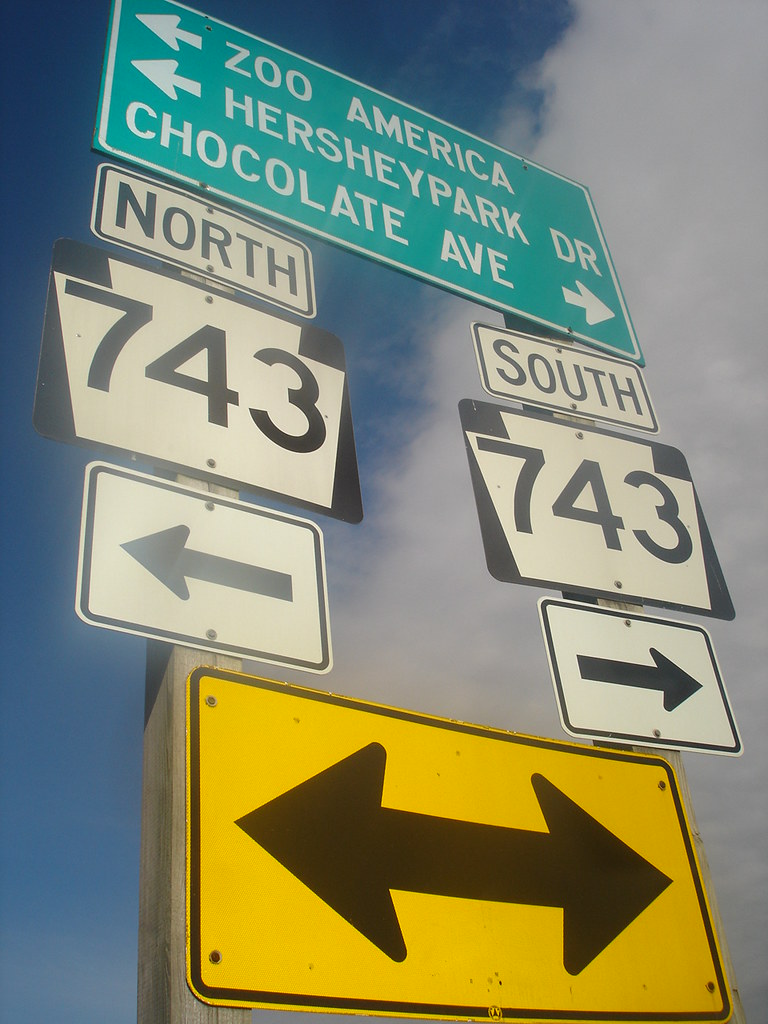This photograph showcases a detailed close-up of a multi-directional road sign set against a backdrop of a bright blue sky, partially filled with fluffy white clouds, predominantly on the right side of the image. At the top of the sign, a large green directional sign features three main destinations: 

1. "Zoo America" with a white arrow pointing to the left.
2. "Hersheypark Drive" also with a white arrow pointing to the left.
3. "Chocolate Avenue" with a white arrow pointing to the right.

Below these green signs, on the left, a black and white sign indicates "North 743" with an arrow pointing to the left. On the right, another black and white sign indicates "South 743" with an arrow pointing to the right. At the very bottom, there is a yellow sign with a black border, featuring a two-headed arrow pointing both left and right, possibly indicating that traffic can proceed in either direction. This sign assembly is likely located in Hershey, Pennsylvania, guiding travelers to local attractions and routes.